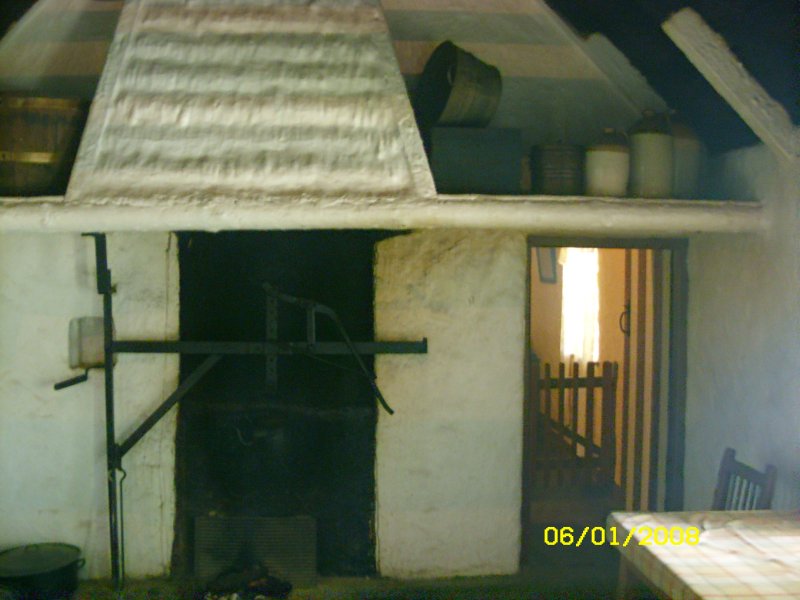This photograph showcases the rustic interior of an old, possibly traditional house, featuring smooth, white plastered mud walls. In the foreground, a table draped with a yellow and white plaid tablecloth occupies the bottom left corner. Above, there are recessed shelves holding baskets and pottery, suggesting an emphasis on storage and simplicity. The right side of the image features a wooden doorway without a visible door, leading to another room with a brown picket fence and is illuminated by sunlight streaming through a window. Another doorway on the left side reveals a dark, unlit space beyond, partially obstructed by a single metal rod contraption. The ambiance reflects a blend of utilitarian design and natural elements, further emphasized by wooden and metal accents. The dated aesthetic suggests the room is from an earlier time, offering a glimpse into traditional living environments.